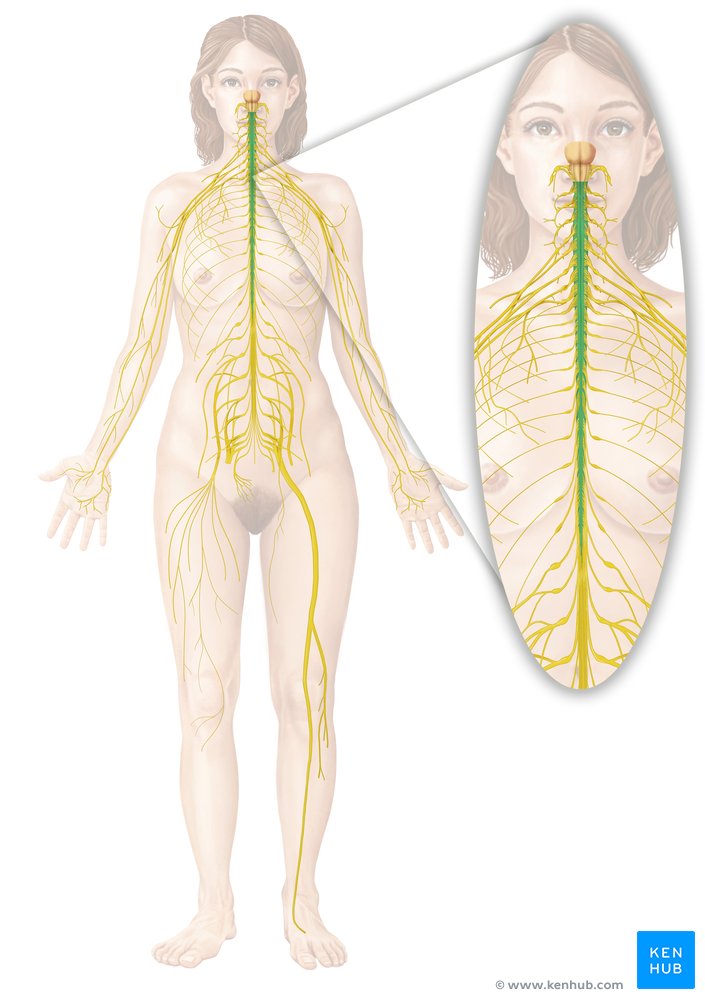The image, sourced from Kenhub (www.kenhub.com) and likely part of a medical publication, features an illustration of a transparently rendered nude woman with shoulder-length wavy brown hair, standing with her palms forward. Overlaying her semi-opaque figure is a detailed depiction of the central nervous system, spinal cord tract, and pathways correlating with embryonic development and the circulatory system. These systems are illustrated with a central green line running from just below the eyes down to the pelvis, branching out into yellow strands that traverse the arms and legs, highlighting the nervous pathways extensively. On the right side of the image, an inset oval magnifies a section of her spinal cord, prominently featuring the same green and yellow detailing. The combination of the main and magnified images offers a comprehensive view of the nervous system's pathways throughout her body.